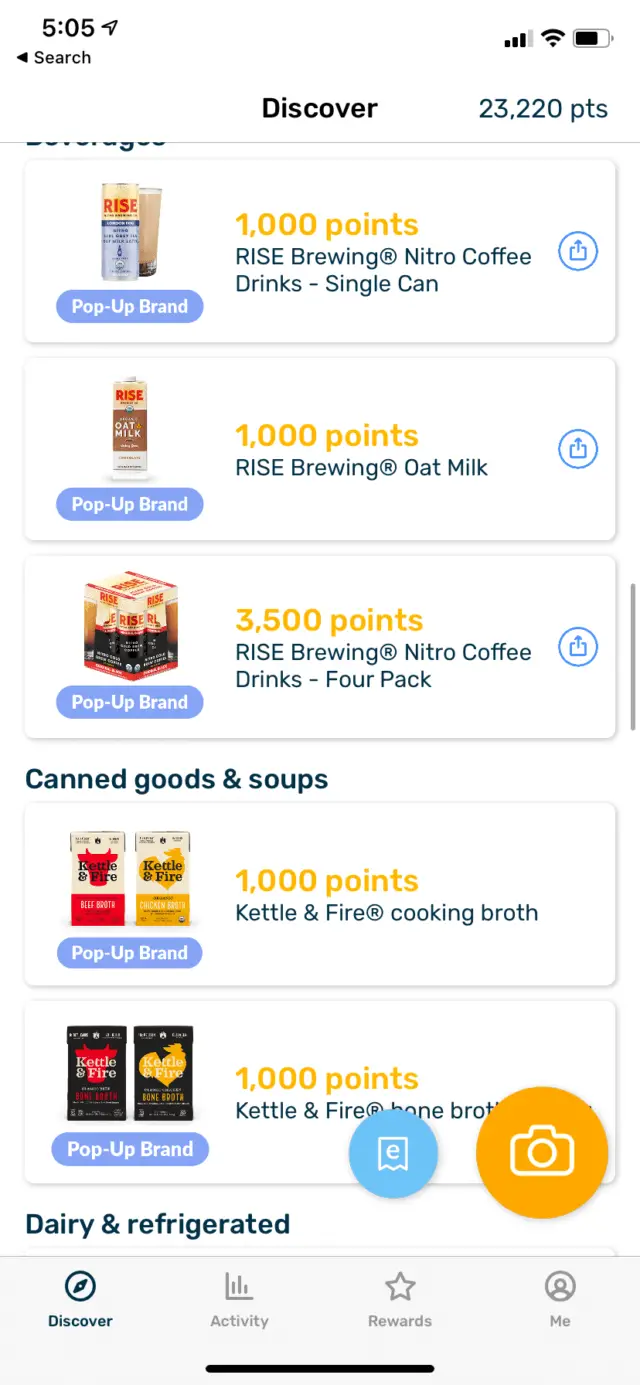Screenshot of a Mobile Shopping App Interface

This detailed screenshot, most likely taken from a phone in portrait mode, showcases a shopping app for food items. The background is a light, slightly off-white color, and the interface is clearly designed for ease of use.

At the top left corner, the current time is displayed alongside a backward arrow. Directly beneath it, small text labeled "search" is accompanied by an arrow pointing left. On the top right, icons show the phone coverage at three out of four bars, a Wi-Fi symbol, and a battery indicator.

Centered just below these indicators, bold text reads "Discover," flanked on the right by "23,220 PTS" in a greenish-blue hue, indicating the user's available points.

The main section of the screen displays five food items, each housed in its own rectangular button:

1. **Rise Brewing Nitro Coffee (Single Can)**:
   - **Points**: 1,000
   - **Category**: Drinks
   - **Label**: "Pop-Up Brand" in a purple rectangle.
   - **Action Icon**: A circle featuring a rectangle with an upward-pointing arrow.

2. **Rise Brewing Oat Milk**:
   - **Points**: 1,000
   - **Category**: Drinks
   - **Label**: "Pop-Up Brand" in a purple rectangle.
   - **Action Icon**: A circle featuring a rectangle with an upward-pointing arrow.

3. **Rise Brewing Nitro Coffee (4-Pack)**:
   - **Points**: 3,500
   - **Category**: Drinks
   - **Label**: "Pop-Up Brand" in a purple rectangle.
   - **Action Icon**: A circle featuring a rectangle with an upward-pointing arrow.

Beneath these, a new heading "Canned Goods and Soups" appears:

4. **Kettle and Fire Cooking Broth**:
   - **Points**: 1,000
   - **Label**: "Pop-Up Brand" in a purple rectangle.
   - **Description**: Cooking broth.
   - **Action Icon**: A circle featuring a rectangle with an upward-pointing arrow.

5. **Kettle and Fire Bone Broth**:
   - **Points**: 1,000
   - **Label**: "Pop-Up Brand" in a purple rectangle.
   - **Description**: Partly obscured by a camera icon in a yellow circle and a blue circle with an "E" inside, encapsulated in a torn paper design.

The bottom-most section visible shows the beginning of a new category titled "Dairy and Refrigerator," though specific items are cut off by a menu bar. This menu bar, located at the very bottom, features four tabs:

- **Discover**: Highlighted in green with a compass icon.
- **Activity**: Grayed out with a graph icon.
- **Rewards**: Grayed out with a star icon.
- **Me**: Grayed out with a circle containing a person's head icon. 

This snapshot provides a clear insight into the app’s layout and functionality, emphasizing ease of navigation and a points-based purchasing system.